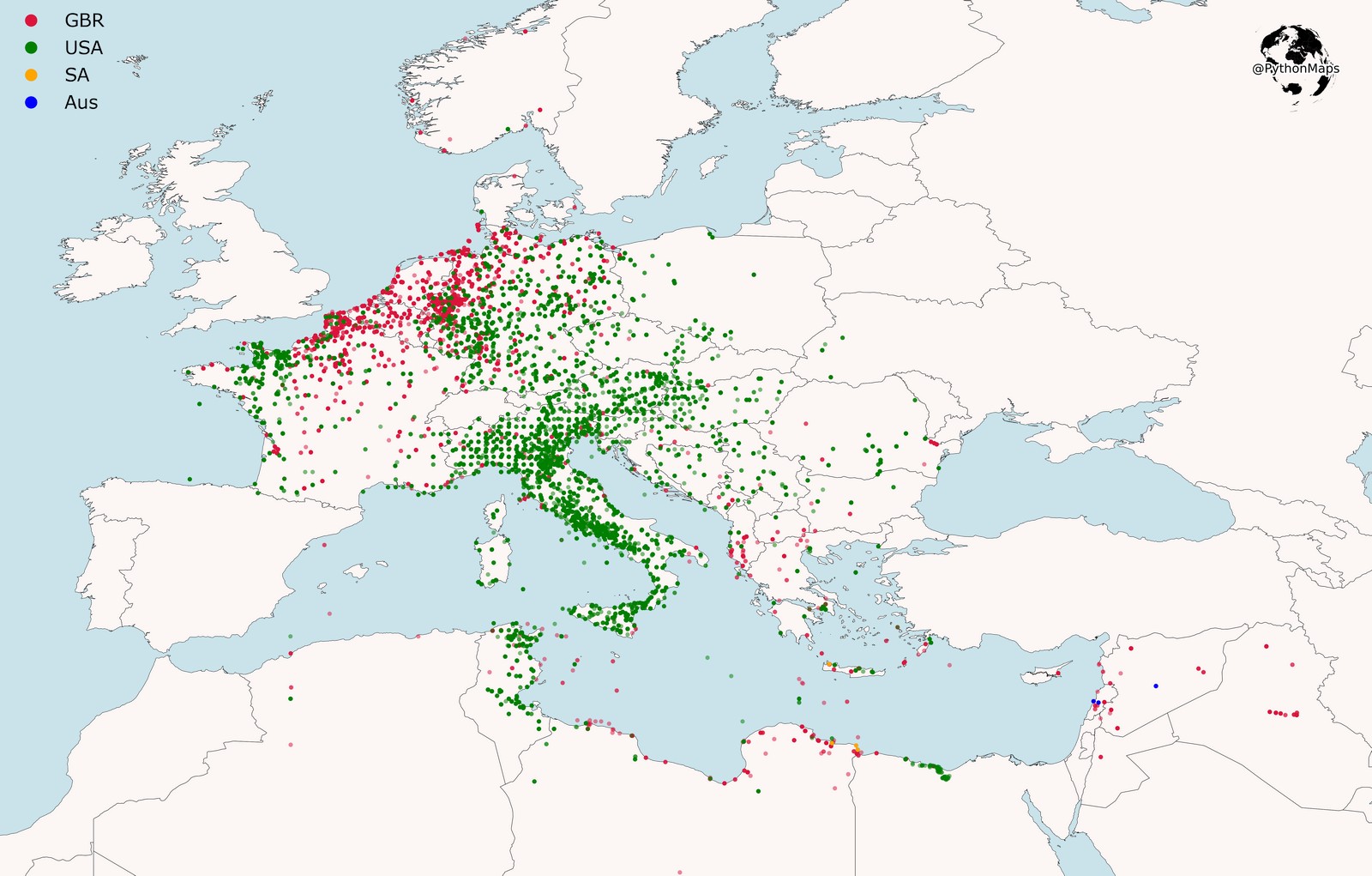The image portrays a detailed map focusing on the Mediterranean Sea, parts of the Atlantic Ocean, Europe, Northern Africa, and the Middle East. The majority of the ocean is depicted in a baby blue color, while the landmasses are mostly white. Distinct areas are marked by colored dots: red for GBR (Great Britain), green for USA, yellow for SA (South America), and blue for AUS (Australia). The upper left corner features a sequence of these dots—red, green, yellow, and blue—with corresponding labels. Notably, green dots (USA) densely cover Italy and Sicily, while red dots (GBR) are concentrated in Northern and Western Europe. Additionally, a significant black globe-like symbol is located at the top right. The map also features a network of lines delineating territorial divisions.